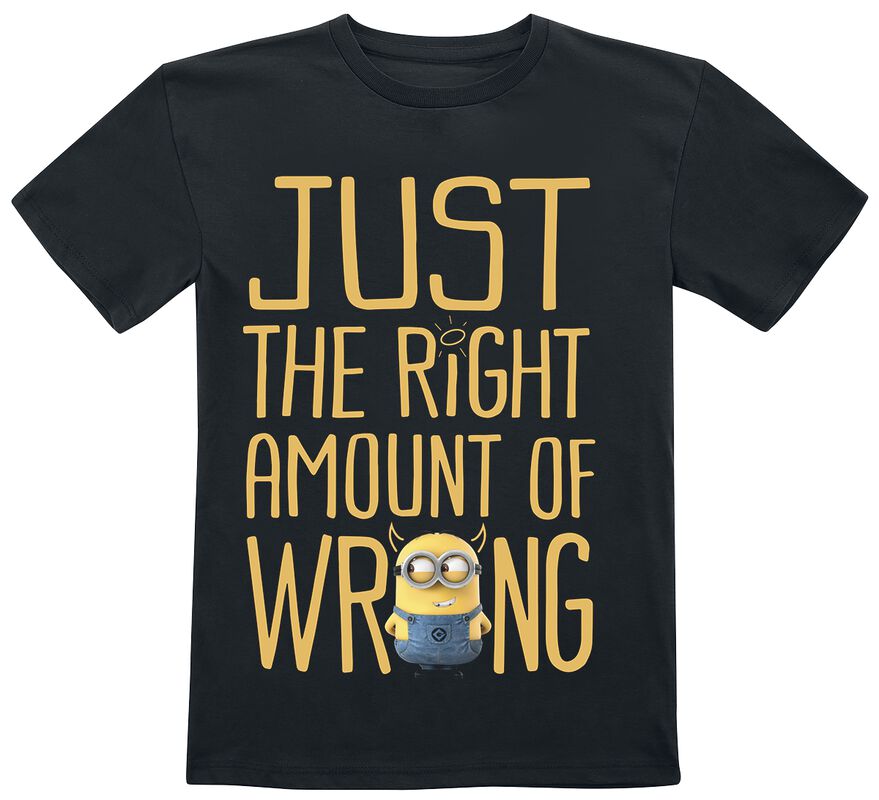The image showcases a black short-sleeve t-shirt laid flat against an all-white background, typical of product display photos on clothing websites. The t-shirt, with a simple crew neck and no fancy stitching, features a prominent graphic design that occupies most of its front. In yellow lettering, it reads, "Just the right amount of wrong." Notably, the dot on the ‘i’ in “right” is depicted as a small circular halo with radiating lines. The 'o' in "wrong" incorporates a playful Minion from the Despicable Me series, who is wearing blue overalls and silver goggles, with drawn-on horns adding to his mischievous look. The Minion, with his eyes shifting slyly to the left and hands behind his back, stands at the bottom of the shirt, adding a whimsical touch to the design. The shirt itself dominates the photo, emphasizing its humorous and visually engaging style. The colors in the design include various shades of yellow, light blue, brown, and the black of the t-shirt, creating a vivid yet cohesive look.